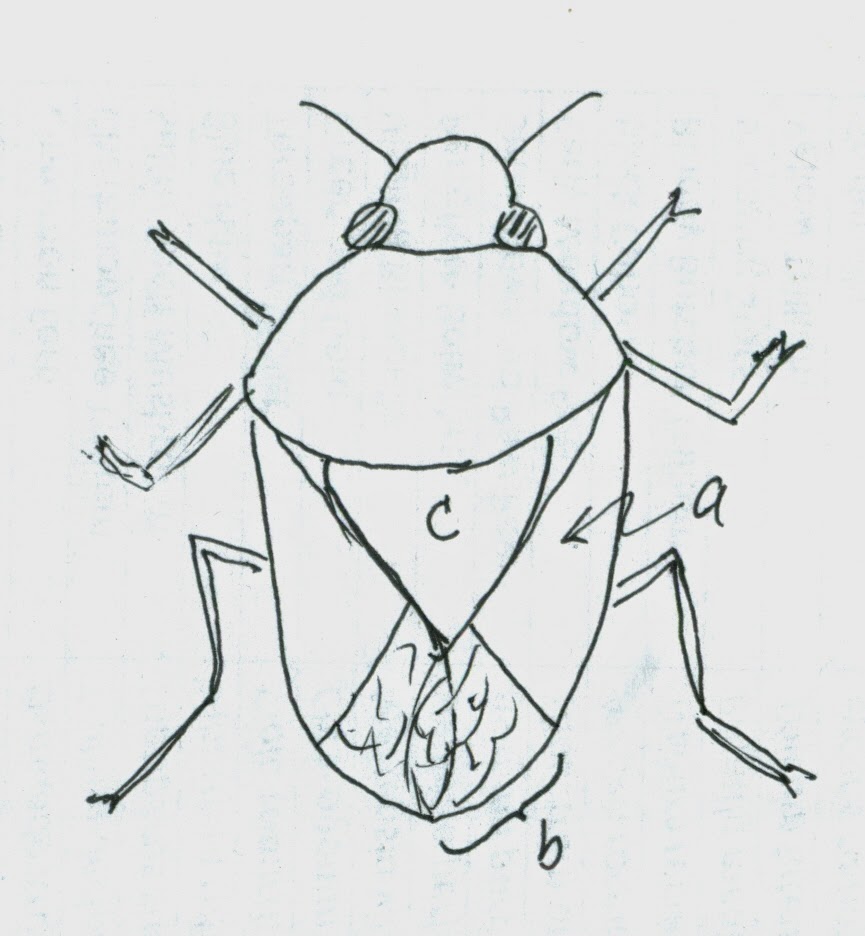This image is a detailed, hand-drawn sketch of an insect, likely a beetle, rendered in black pen on white paper. The body of the beetle is divided into various segments labeled A, B, and C, though there is no explanation for these labels. Segment A is situated on the right side, B is on the back, and C is in the middle of the insect. The drawing is primitive but precise, with minimal shading on the back, eyes, and one leg. The beetle's anatomy is clearly illustrated, featuring six legs positioned in various orientations: straight legs near the top, V-shaped legs in the middle, and upside-down V-shaped legs at the bottom. The insect has two prominent antennae and eyes located on each side of its head. The background is a solid light gray with faint, vertically aligned printed text visible from the opposite side of the paper. Despite the simplicity and lack of color, the drawing effectively captures the main anatomical features of the beetle, demonstrating the artist’s skill and attention to detail.